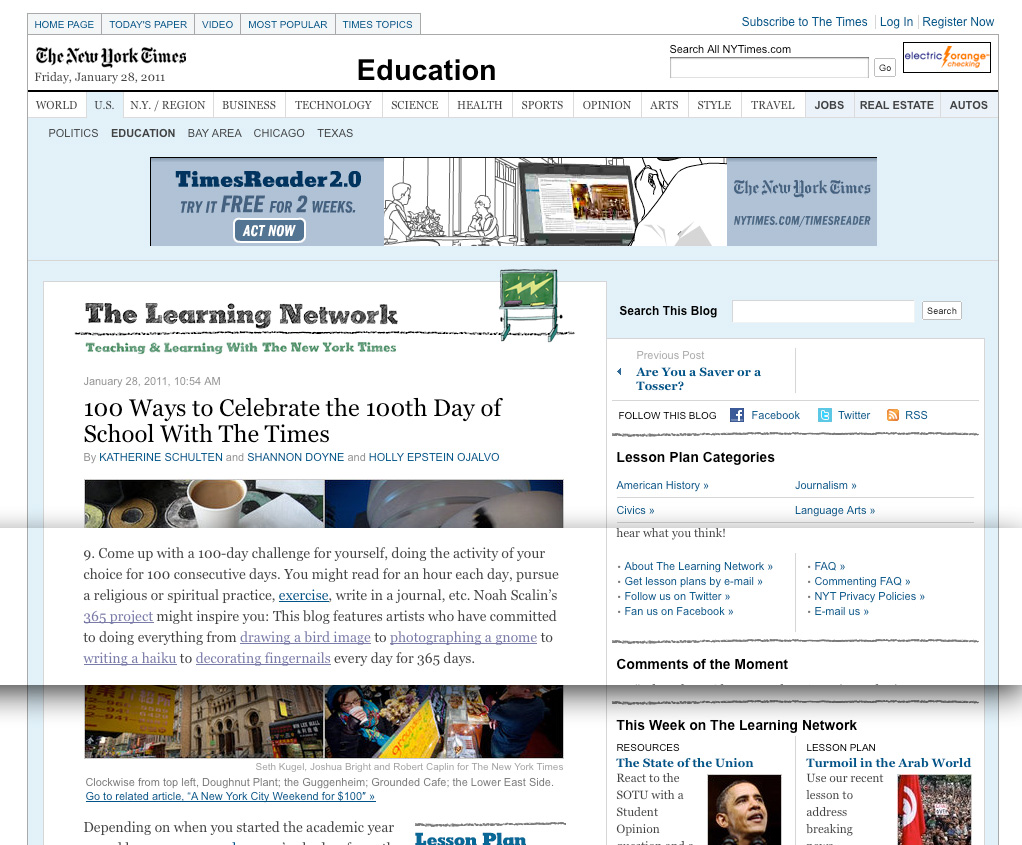This is a detailed description of a page from The New York Times website as it appeared on Friday, January 28, 2011. The upper left-hand corner features a light gray navigation bar with bright blue text, providing tabs for various sections including "Homepage," "Today's Paper," "Video," "Most Popular," and "Times Topics." On the far right, users find options in bright blue text to "Subscribe to the Times," "Log In," or "Register Now."

Directly beneath this navigation bar, the iconic "The New York Times" logo is displayed prominently in its traditional black font. Below the logo, the date "Friday, January 28, 2011" is noted. Centered on the page, the word "Education" is boldly printed in black type, indicating the focus of the content on this particular section.

To the right of the "Education" heading, there is a search bar labeled "Search All NewYorkTimes.com." Below this, an additional navigation bar stretches across the page with tabs for specific sections including "World," "U.S." (which is currently selected), "New York Region," "Business," "Technology," "Science," "Health," "Sports," "Opinion," "Arts," "Style," "Travel," and further options like "Jobs," "Real Estate," and "Autos" on the right. 

Further down, a secondary navigation menu in gray text lists "Politics," "Education," "Bay Area," "Chicago," and "Texas." Below this menu, there is an advertisement for "Times Reader 2.0," featuring navy blue text on a light purple background and a promotional offer to "try it free for two weeks." A gray button with a white border labeled "Act Now" in white text accompanies this ad.

At the bottom of this section, "The Learning Network" is printed in bold black text, followed by the tagline "Teaching and Learning with the New York Times," emphasizing resources available for educators and students.